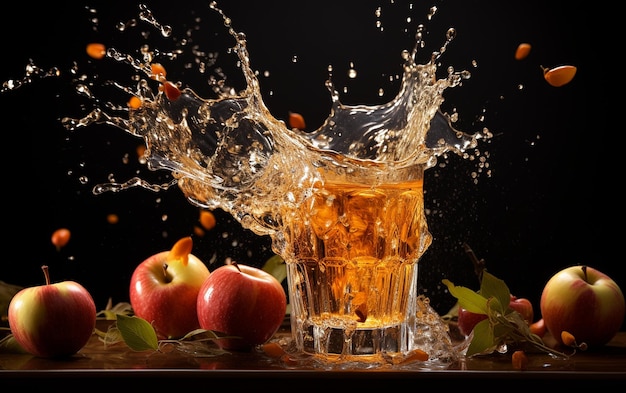In this color photograph, a clear transparent drinking glass filled with a liquid the color of apple juice or light amber apple cider is captured mid-splash. The splash is dramatic, with the liquid rising and spilling over the top of the glass, reminiscent of the explosive effect when something is dropped in. The background is a solid, deep black, which makes the splash and liquid stand out vividly. Surrounding the glass on its left and right, several red and green apples are placed on a shiny, reflective surface, enhancing the scene's freshness. Among the apples and the splash, small red round objects, possibly cherry tomatoes or flower petals, add an element of intrigue—perhaps one was the trigger for the splash. Some green leaves also adorn the surface, likely apple leaves, suggesting the apples are freshly picked. The overall scene evokes a sense of refreshing sweetness and ripe abundance.